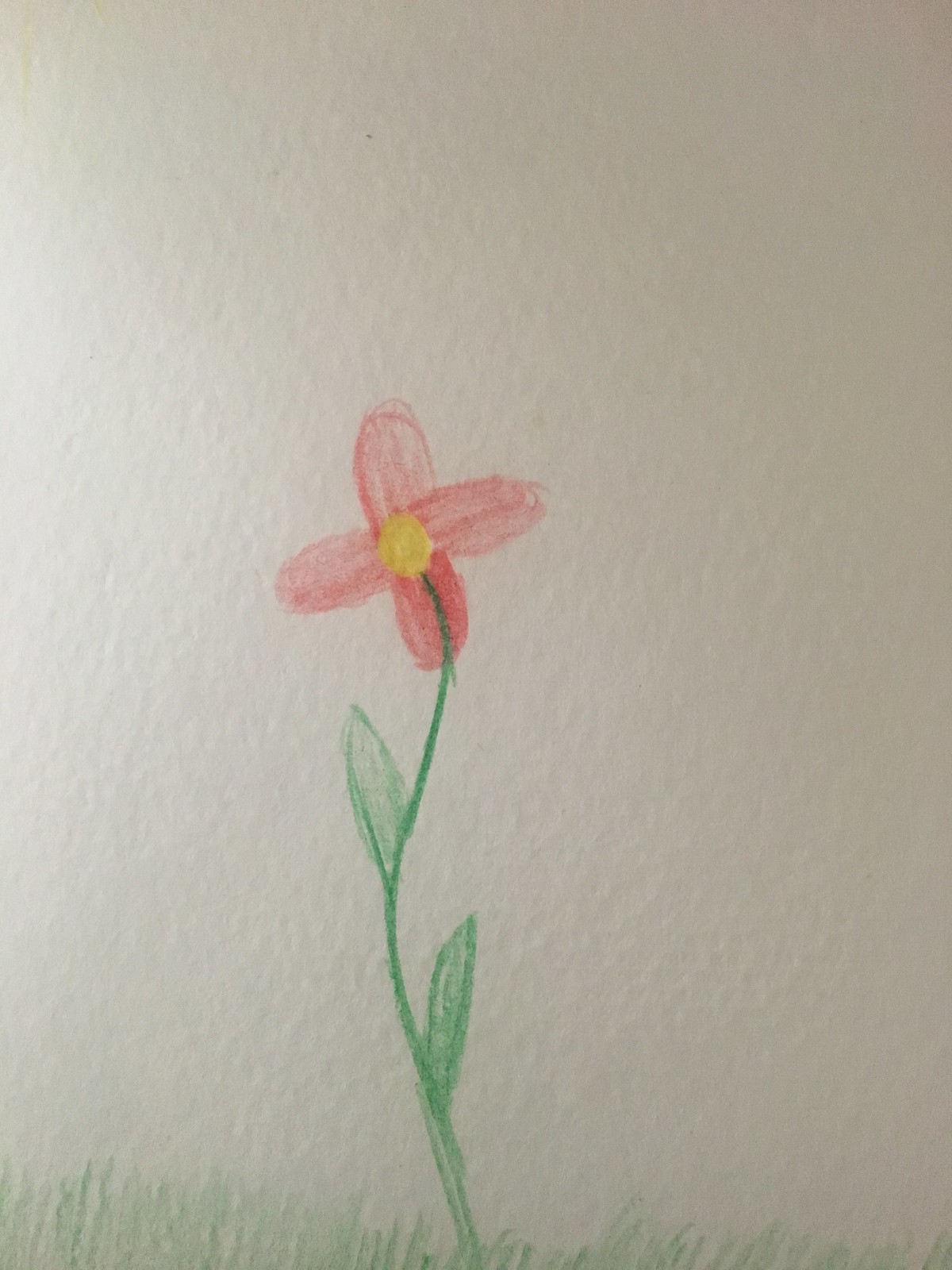This vertically aligned portrait-style image captures a simple and charming drawing of a flower, rendered meticulously in crayon or colored pencil on a piece of thick white or slightly off-white drawing paper. The solid white background contrasts beautifully with the vibrant colors of the drawing, emphasizing its child-like essence.

At the bottom of the image is a small patch of straight green grass from which a slender, slightly curving green stem rises. The stem features two small leaves, one on each side. Crowning the top of the stem is a four-petal flower, depicted in shades of pinkish-red to dark pink, complete with a yellow, bulb-like center.

While the flower and its surroundings demonstrate a simplicity often seen in children's artwork, the image is filled with small details: the textured paper, the overall neat coloring, and the striking contrast between the flower's bright petals and the plain backdrop. This composition elegantly highlights the charm and innocence of a child's creative expression.